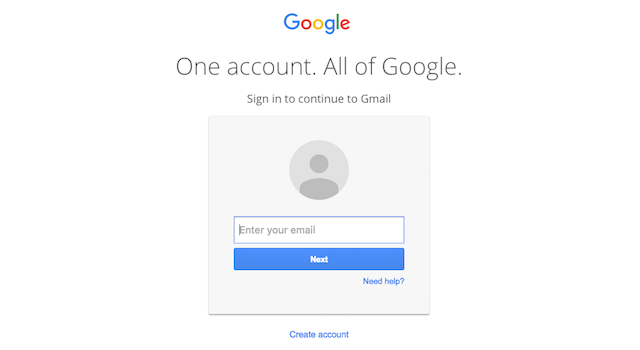The image depicts a clean, minimalistic Google sign-in screen. At the top, the iconic Google logo is prominently displayed with each letter in its respective color: the first 'G' in blue, the 'o's in red and yellow, the second 'G' in blue, the 'l' in green, and the 'e' in red. Beneath the logo, a headline reads, "One account. All of Google." Below this, a subheading prompts users to "Sign in to continue to Gmail."

The central portion of the screen features a placeholder icon resembling a generic person, indicating where users should enter their email address. Adjacent to the icon is a text field labeled "Enter your email." Below this input box is a blue button labeled "Next," and underneath that are links for "Need help?" and "Create account." The overall design is straightforward and uncluttered, focusing solely on facilitating user login to access Google's services, specifically Gmail. The absence of additional images or distractions reinforces the simplicity and user-friendliness of the login process, guiding users step-by-step to enter their email and proceed to the next stage, which likely involves password entry.